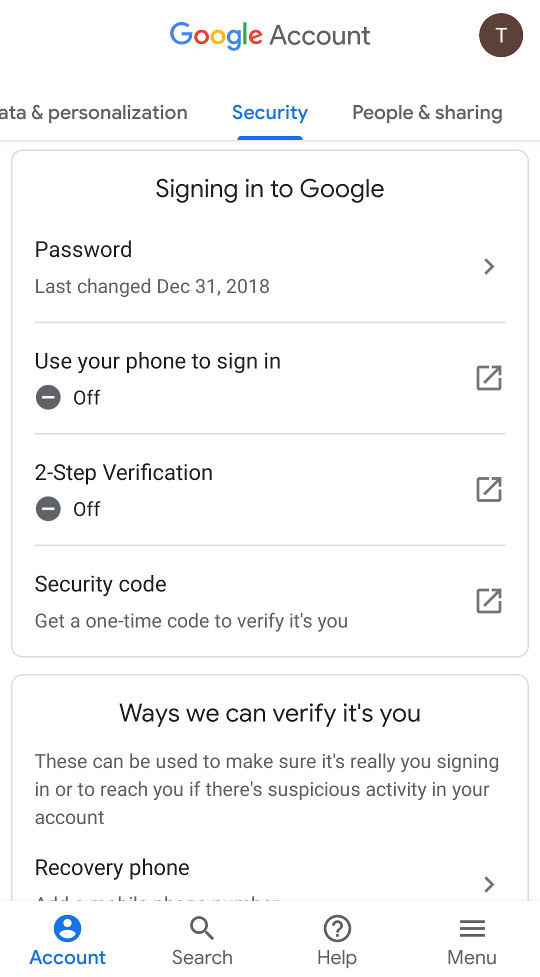This image is a cropped mobile screenshot displaying the Google Account settings page. At the top center, the heading "Google Account" is visible, and in the top-right corner, there is a profile picture represented by a capital "T". Beneath the heading, various scrollable categories are listed, with the "Security" category highlighted in blue at the center of the screen.

The main content area showcases a large white box titled "Signing in to Google", centered at the top of the box. This section features a vertical list of security options. The first item in the list is "Password", accompanied by a date indicating the last change, and an arrow pointing to the right. Following this, there is an option labeled "Use your phone to sign in", which is marked as off. Below that is "2-Step Verification", also noted as off. At the bottom of this list, there is "Security Code" positioned to the left.

Underneath the "Signing in to Google" box, there is a smaller box titled "Ways we can verify it's you", centered at the top. A brief description follows, explaining that these methods can be utilized to confirm your identity during sign-in or to reach you in case of suspicious activity. The first item listed under this section is "Recovery Phone", but the specific information related to it is not visible in the screenshot, indicating that additional scrolling would be required to view this data.